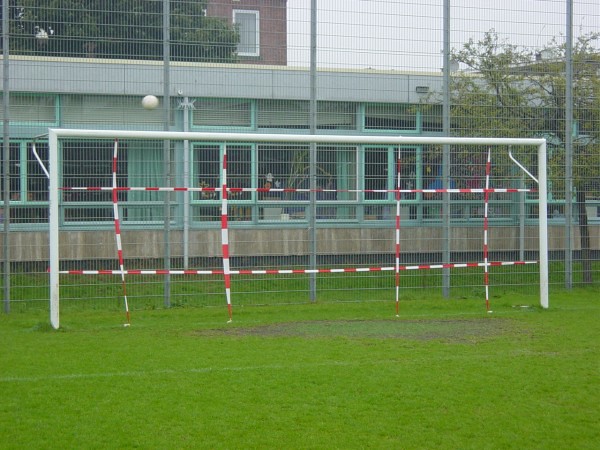The image depicts an outdoor play area in front of what appears to be a school building. The foreground features a partially visible soccer pitch with a white goalpost. The goalpost has a red and white danger or keep-out pattern on its frame, comprising two horizontal and four vertical bars. The pitch itself is covered in green grass. Behind the goalpost and pitch, there is a tall metal fence supported by five vertical poles with wires running horizontally. The school building beyond the fence has light green window trims, green curtains, and decorations taped onto the windows. Additionally, a plant is visible growing in the second window from the left. The building's exterior includes gray and reddish brick elements. The sky is cloudy, and there are trees on both the right side and behind the fence, with varying shades of green leaves.